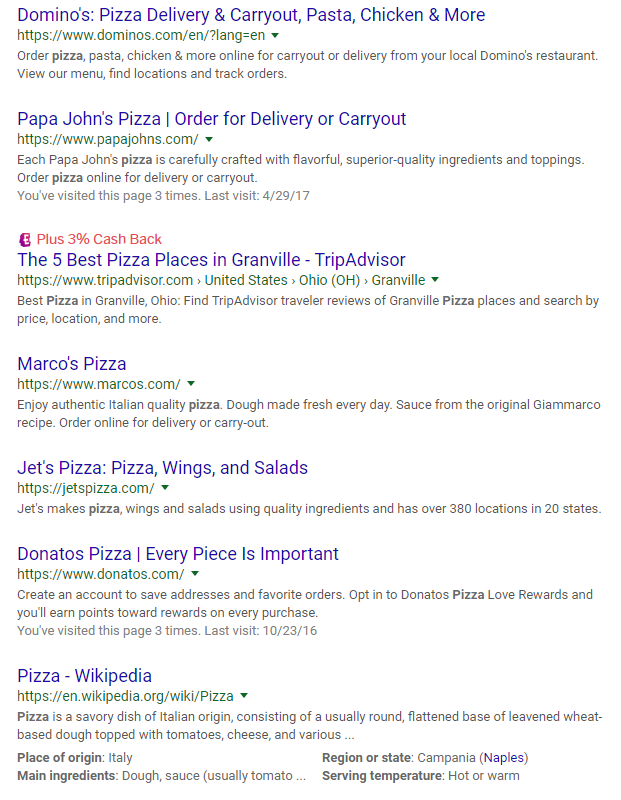In this image, a search results page for various pizza locations and restaurants is displayed. The search query has yielded seven results, each highlighting different pizza places and information. The first result is "Domino's Pizza," offering delivery and carry-out options along with their menu items like pasta and chicken. The second result features "Papa John's Pizza," also providing delivery and carry-out services.

Following these, the third result is a Trip Advisor listing titled "The Five Best Pizza Places in Granville." The fourth search result is for "Marco's Pizza," while the fifth highlights "Jert's Pizza," which offers pizza, wings, and salads. The sixth result showcases "Donato's Pizza," with the tagline "Every piece is important."

The final search result leads to a Wikipedia page about pizza, detailing that pizza is a savory dish of Italian origin. It traditionally consists of a usually round, flattened base made from leavened wheat dough, topped with tomatoes, cheese, and various other ingredients. The description also mentions that its place of origin is Italy, specifically pointing out the regions of Campania and Naples as significant.